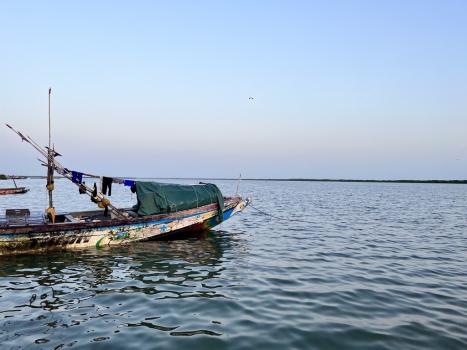The image portrays a vast, dark, and almost smooth expanse of water, echoing the look of Southeast Asia with its barely visible, flat, distant shoreline under an overcast bluish-gray sky. In the left side of the image, an old, narrow, and heavily beaten-up boat rests. This boat, possibly a fishing vessel or living quarters, shows signs of severe wear and tear. Its sides are scuffed and scraped, with the hull appearing burnt. A torn sail hangs in shreds, and a green tarp at the bow indicates a makeshift sleeping area, with pants and other clothing items hung over a stick. The boat conveys a sense of abandonment, floating eerily in the water without any visible inhabitants. In the distance, there is another boat or perhaps a dock barely peeking out from the left side of the frame.